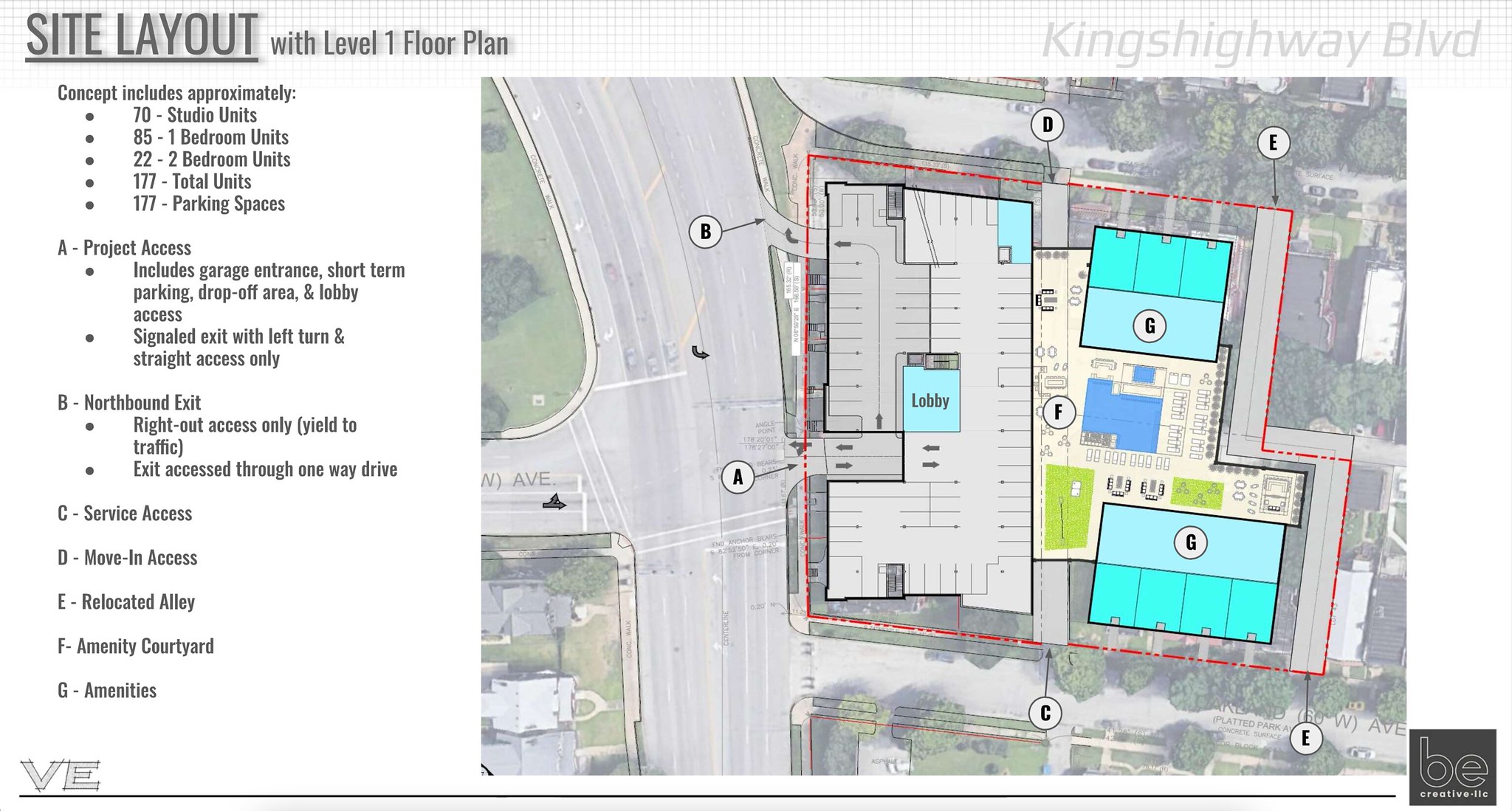The image is a detailed site layout of a large building project, featuring a level one floor plan. The concept includes approximately 70 studio units, 85 one-bedroom units, and 22 two-bedroom units, totaling 177 units and 177 parking spaces. The layout shows project access with a garage entrance, a short-term parking and drop-off area, lobby access, and a signaled exit limited to left turns and street access only. Key features include a northbound exit with a right-out access that yields to traffic and exits through a one-way drive, service access, move-in access, a relocated alley, an amenity courtyard, and various other amenities.

The illustration is a bird's-eye view rendered as a black-and-white line art overlay on an aerial photograph, with spot color applied for emphasis. The map is predominantly on the right side, with significant annotations labeled A through G: 
A - Project access
B - Northbound exit
C - Service access
D - Move-in access
E - Relocated alley
F - Amenity courtyard
G - Amenities

The map is bordered by King's Highway Boulevard on the top right, with abbreviations VE and BE located in the bottom left and right corners, respectively. The graphic elements use condensed black text and colored illustrations to highlight various aspects of the site layout, providing a comprehensive and visually informative overview of the planned development.